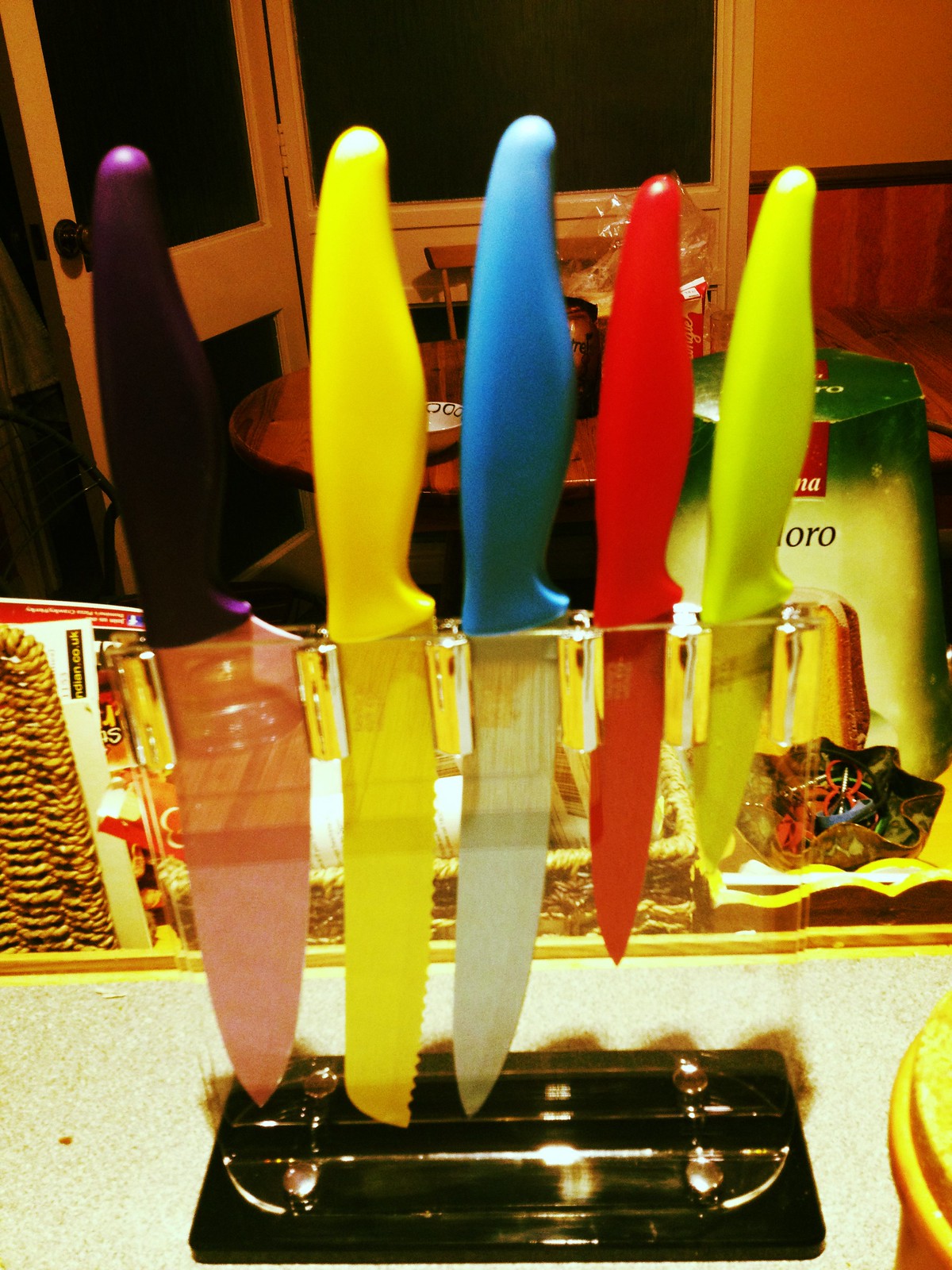In this photograph of a kitchen setting, a vibrant set of five knives is prominently displayed in the foreground. The knives are neatly arranged side by side in a clear, Lucite knife block with a black base, which makes the colorful handles and blades stand out. From left to right, the knives decrease in size: the first knife on the left is the largest with a black handle and a purple blade. Next is a large serrated bread knife with a yellow handle and blade. The third knife has a blue handle and silver blade, followed by a smaller paring knife that's entirely red. The smallest knife on the right has a lime green handle and blade. 

Behind the knife block, the setting features a kitchen countertop, possibly made of granite, with various kitchen items: a wicker basket filled with papers, a can with an obscured label ending in “NA” and “ORO,” and a bag of what appears to be a small cake. In the background, there is a round wooden table with two wooden chairs, a white bowl on the table, and a doorway framed in yellow next to a window. The room has wood paneling, adding a rustic touch to the overall scene.